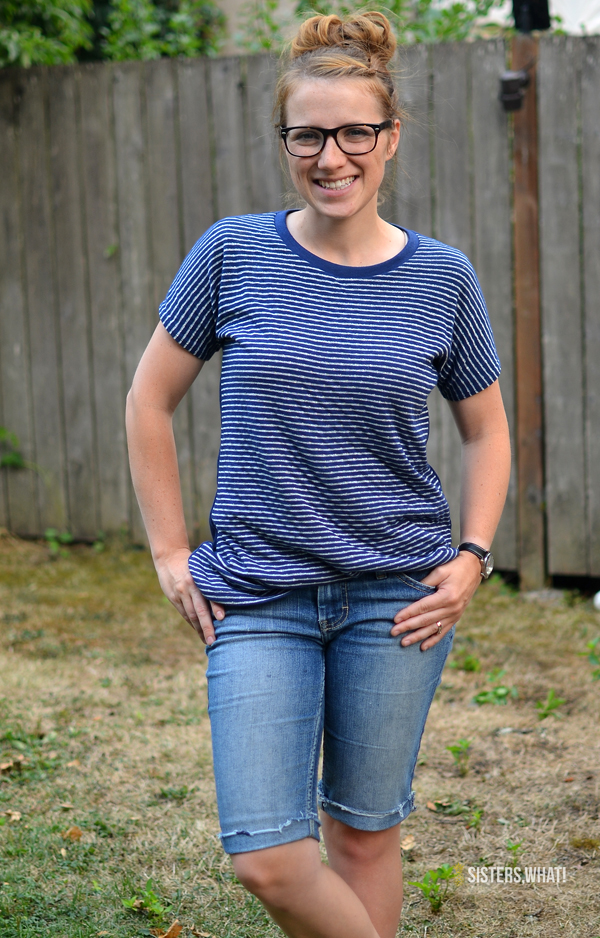A woman is seen smiling broadly at the camera in an outdoor setting, likely in a backyard. She is a Caucasian female with dirty brown hair tied up in a bun, wearing black glasses. Her attire includes a blue and white horizontally striped shirt paired with faded blue jean shorts, and a black wristwatch on her wrist. She stands with her hands in her pockets, facing directly toward the viewer. The photo captures her from head to about halfway down her calves. In the background, there is a dark grayish-brown wooden fence with the tops of trees visible above it. The ground she stands on is a patchy, predominantly brown yard with sparse, low weed growth. The overall scene suggests a bright day, and there is a watermark at the bottom right that reads "Sisters What!"